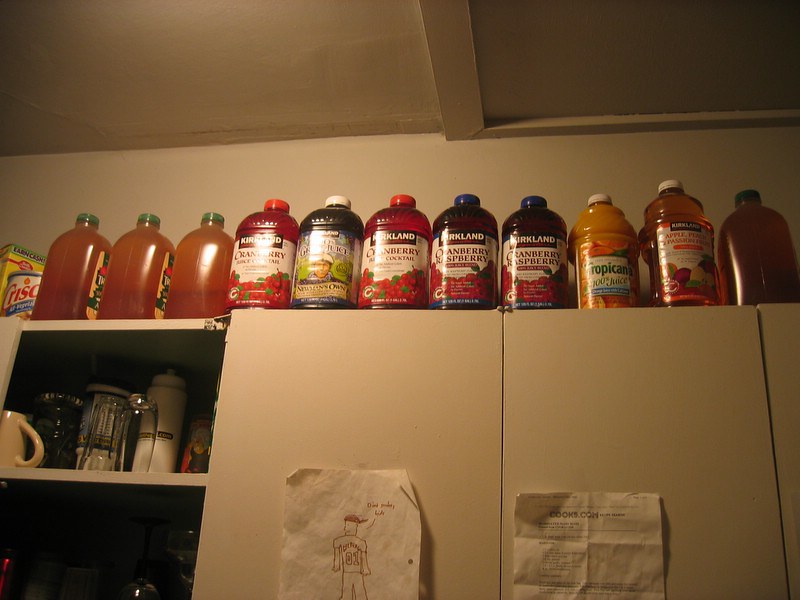This image depicts a dimly lit dry goods storage area within a home, likely a kitchen, revealing a prepper-type setup for long-term storage. The focus is on the top shelf of a set of built-in white cabinets. Illuminated by light from above, we see several drink bottles neatly arranged in a row. Contained on top of the cabinets are brand-new, unopened bottles, including Kirkland cranberry raspberry juice, cranberry juice cocktail, Tropicana juice, and apple juice. There are about eight bottles, with most labels facing forward while a few are turned sideways.

Below the shelf, there are three closed cabinets to the right and one open cabinet to the left, the latter revealing a collection of coffee cups, tumblers, and glasses. Two pieces of paper are taped to the cabinet doors: one is a drawing, and the other appears to be a recipe from cooks.com. The overall scene has a slightly warm, dim tone, and a mix of a homey yet utilitarian atmosphere, emphasizing the organized storage of essential items.